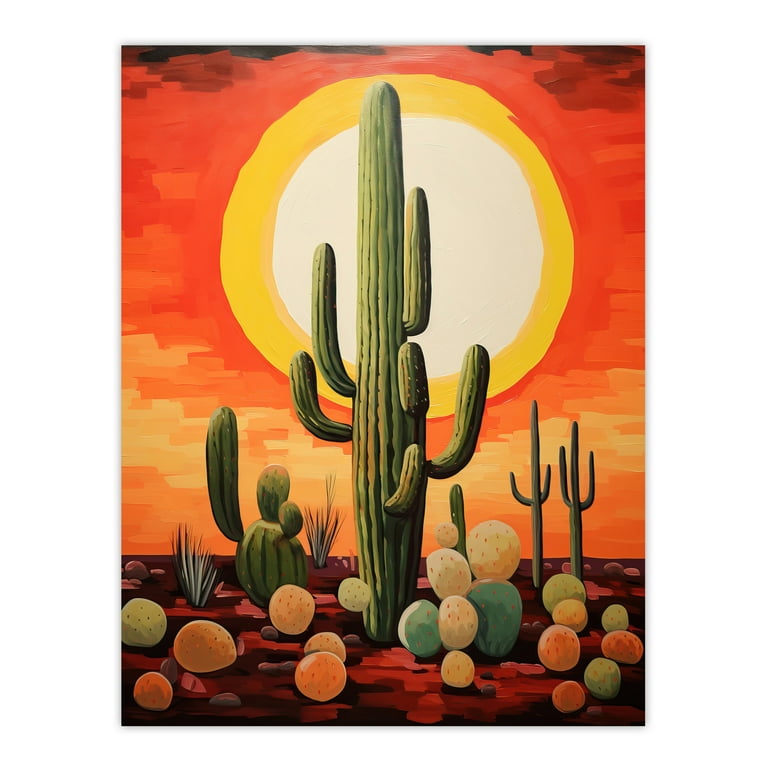The image is a vibrant and detailed painting, possibly a watercolor or computer-generated artwork, featuring a large green cactus prominently in the center, with about five or six arms stretching out. Surrounding this main cactus are several smaller cacti, creating a clustered desert scene. At the cactus's base lie numerous circular objects in shades of pink, green, off-white, orange, light yellow, and blue, which could be futuristic-looking rocks or succulent-like formations, resting on a reddish-colored ground. Behind the central cactus, a striking sun is partially visible, characterized by a white core encircled by yellow. The sky transitions from a darker orange at the top to a lighter orange near the horizon, suggesting a sunset backdrop. The overall scene is vividly depicted, with a rich palette of colors enhancing the desert's surreal and possibly futuristic atmosphere.